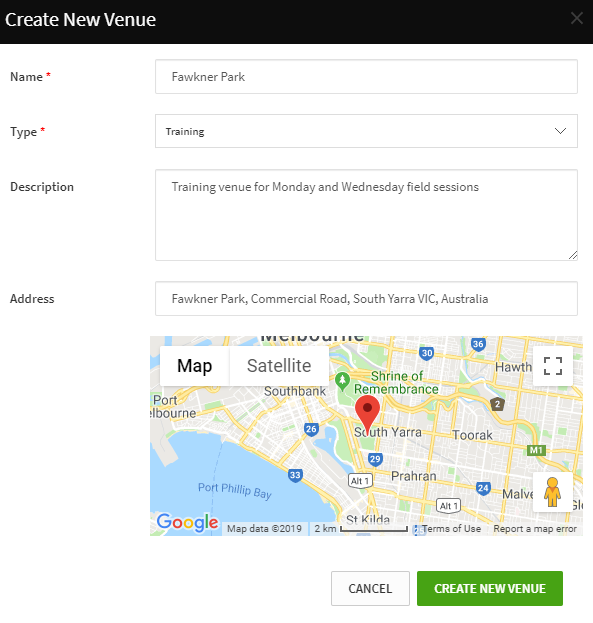At the top of the interface, there is a black horizontal band with white text that reads "Create New Venue" positioned on the left. Below this, the first field is labeled "Name" with a red asterisk indicating it's a required field. The input box next to this label is filled with the text "Fowler Park," with an alternative spelling in parenthesis, "F-A-W-K-N-E-R Park."

The next section is labeled "Type," also marked with a red asterisk to denote its mandatory nature. This field includes a dropdown menu with "Training" selected. Accompanying this is a description detail: "Training venue for Monday and Wednesday field sessions." 

Following this is the "Address" field, pre-filled with "Faulkner Park, Commercial Road, South Y-A-R-R-A-V-I-C, Australia." 

Beneath these input fields, a Google Map is displayed showing the location marked with a red pin. The map features a variety of colors including blue, yellow, green, gray, and white for different landscape elements. In the bottom right corner of the map, there is a small orange figure icon, which typically represents Google Street View.

At the very bottom of the interface, there are two buttons: a white "Cancel" button with black text, and a green "Create New Venue" button with white text.